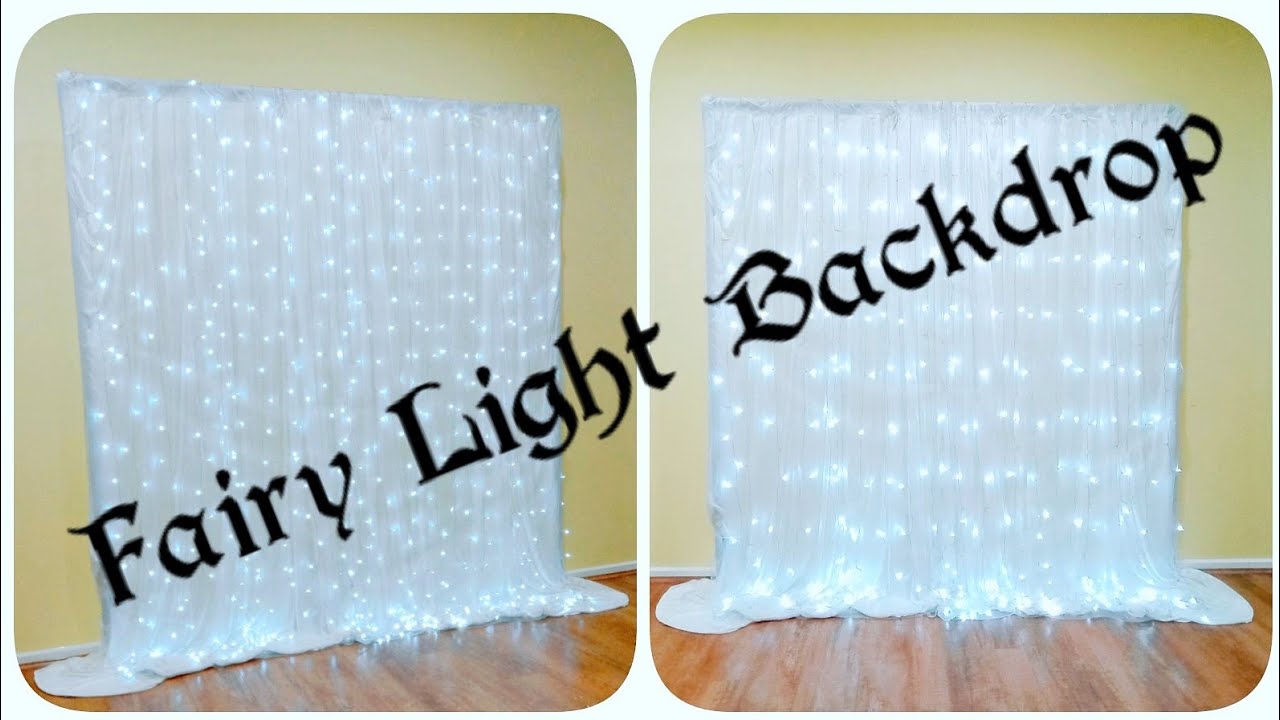The image features two side-by-side photos of a "Fairy Light Backdrop," with this text prominently displayed in bold, black letters across both pictures. Both images showcase the same scene from slightly different angles; one is head-on while the other is taken at a slight angle. The setting includes pale yellow walls and subtly shiny, dark brown wooden floors, with a small white strip separating the wall from the floor. In each image, blue specks of light, possibly from small LEDs or fairy lights, create a glowing effect on what appears to be white sheets or drapes. These little lights also reflect off the wooden floor, adding a grayish hue where they meet the surface. Despite the different perspectives, both photos aim to highlight the fairy light backdrop effectively.